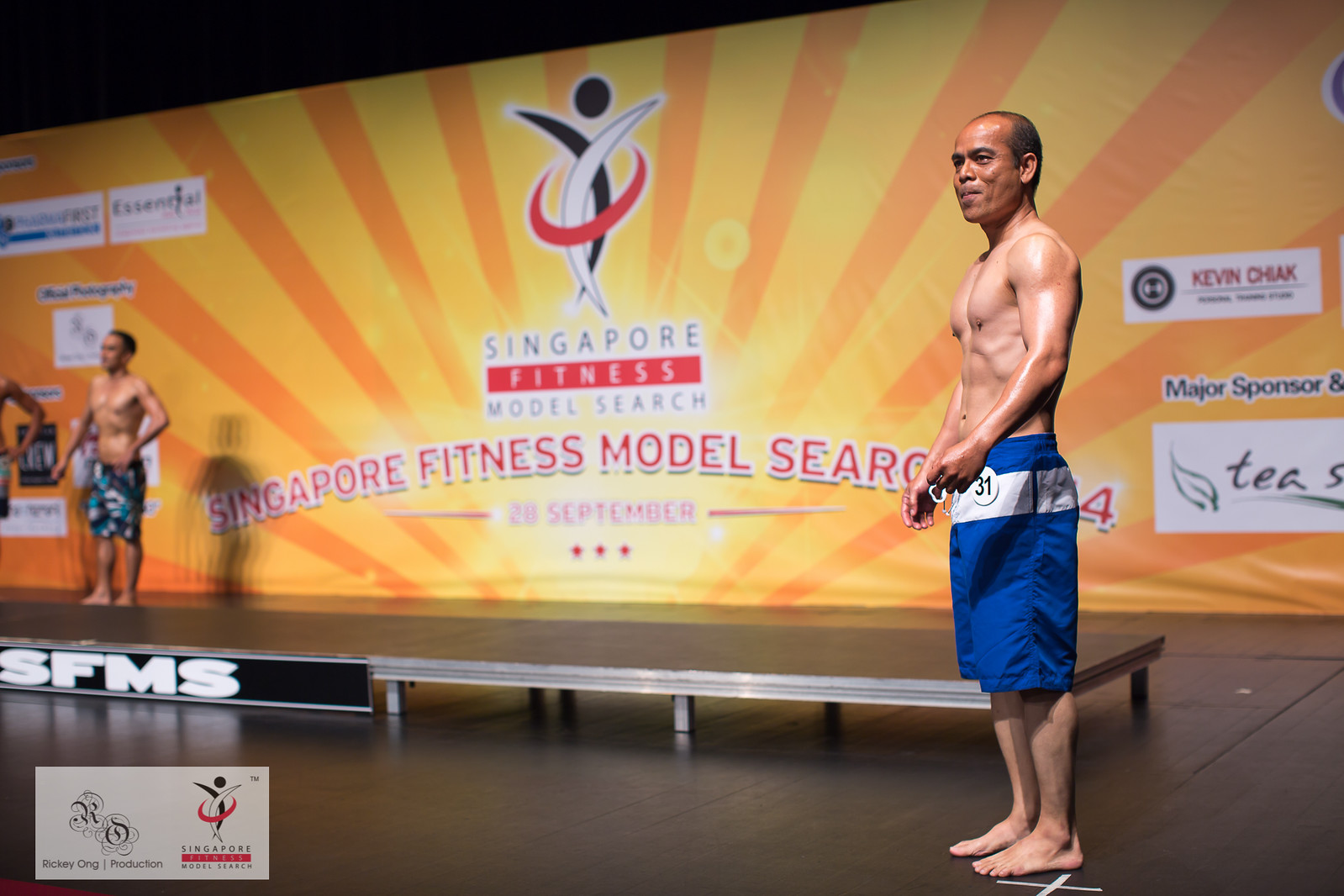In an indoor setting, a shirtless man with dark black hair and a receding hairline stands barefoot and slightly turned towards the center on a stage marked with a white "X." He extends his arms forward, revealing a white ring looped around his ring finger on the visible hand. Clad in blue shorts adorned with a white circle near the waistband featuring a pinned white badge displaying the number "31," the man is accompanied in the distant background by another shirtless individual sporting black shorts with teal and white patches. 

Behind them, an assortment of promotional elements converges into a cohesive scene. A shallow table adorns the left side, emblazoned with "SFMS" in white letters on its bottom surface. Dominating the background, a large banner showcases interconnected circular lines in white, black, and red, anchored by a black circle above them. Radiating sunshine rays span outward to both the left and right sides. Central to the banner's design, "Singapore Fitness Model Search" is boldly repeated, accompanied by the date "20 September" and underscored by three stars. At the banner's lower left corner, another rectangle proclaims "Ricky Org Production" alongside yet another instance of the "Singapore Fitness Model Search."

The overall scene suggests an event centered around a fitness model search, potentially part of a larger marketing or advertising campaign, given the presence of organized signage and the men's prepared, possibly oiled-up appearances. The controlled indoor environment, meticulous labeling, and detailed promotional material all contribute to a vibrant, organized spectacle aimed at selecting or showcasing fitness models.